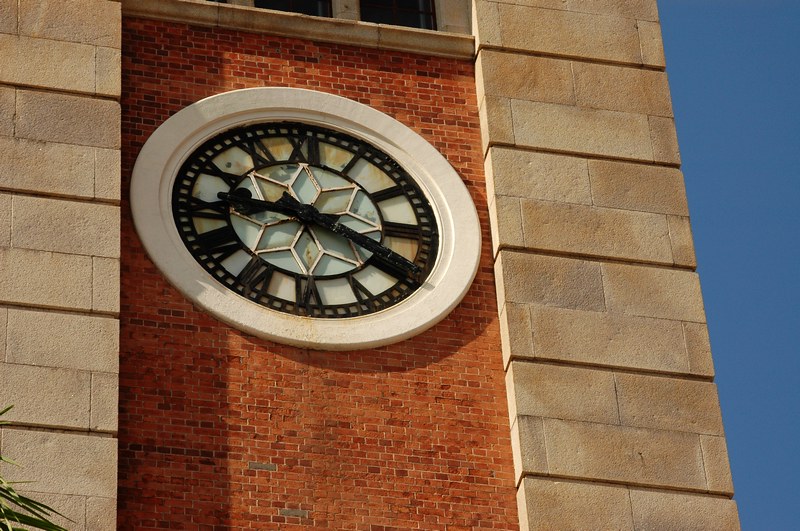This photograph showcases the facade of a brick building, prominently featuring an ornate clock set into what appears to be large brown bricks on the exterior and smaller red bricks visible through the windows. The clock face, resembling a stained glass window, is bordered by a circle of white stone and features heavy, dark Roman numerals from 1 to 12. The clock hands, which are thick and black, are positioned at 9:20. In the center of the clock, light blue, brown, and white triangles form a star pattern, adding to its decorative appeal. To the left bottom corner of the picture, green stalks emerging from bushes or trees are visible. Above the clock, the building extends upwards into what looks like a tower or more windows, with a strikingly clear blue sky framing the right-hand side of the structure.